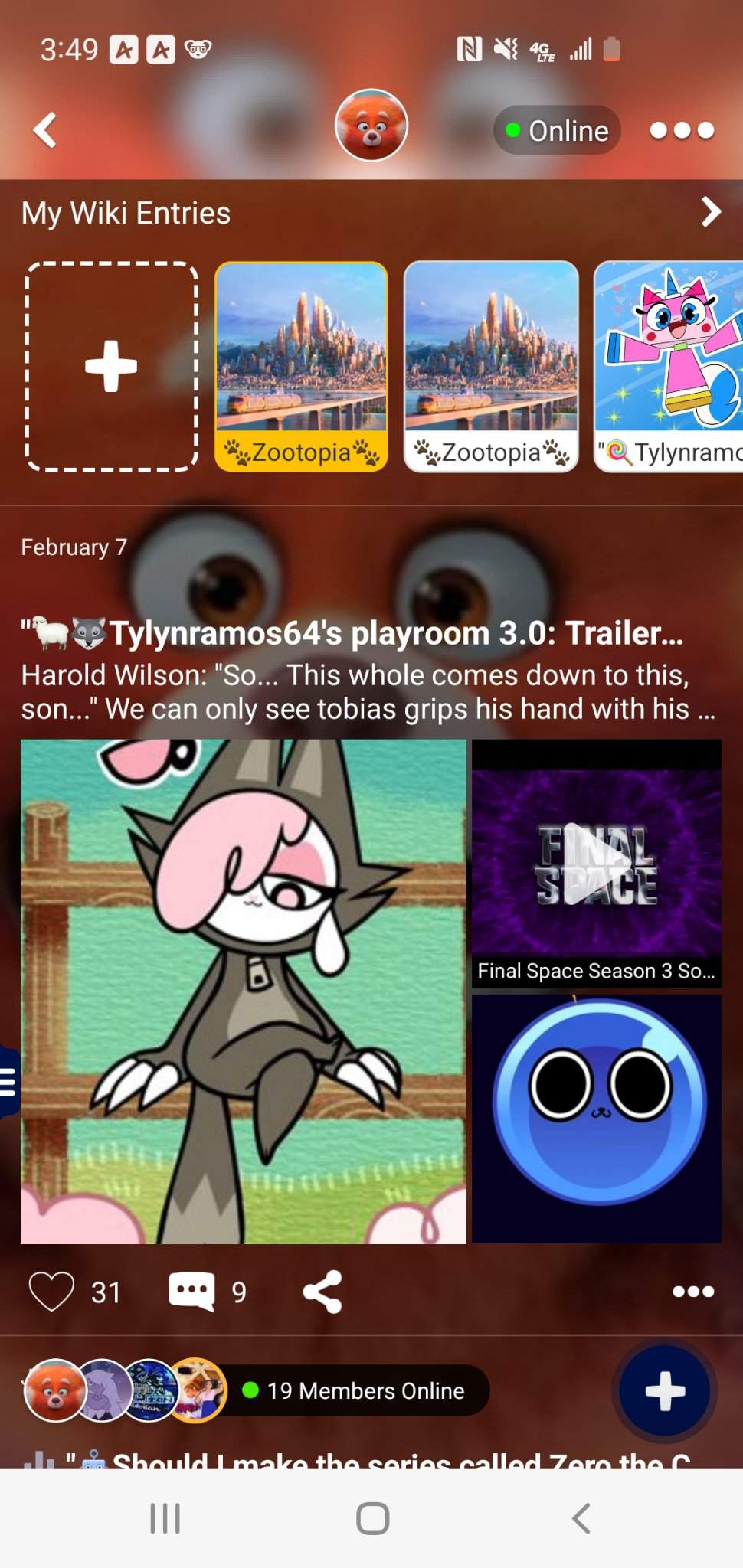The image features a complex and detailed interface with multiple elements on a primarily deep red and darker red background.

At the top of the image, there is a deep red section that displays the number "349" accompanied by a left arrow. Next to it, there is a circle with a small picture of a bear, followed by a button labeled "online" with a small green circle indicating the status.

Below this area, there are three white circles, which transition to a darker red section that bears the text "my wiki entries" along with a right arrow. This is followed by a dotted box containing a plus sign.

In the middle section, there are three small square pictures. The first square, labeled "Zootopia," features a yellow bottom border with four paw prints and an image of a cityscape with a bridge. The second square, also labeled "Zootopia," has a white bottom border. The third square shows a blue background with a small pink character holding what looks like a lollipop, with text partially reading "Talon Ramos."

In another dark red box, one can see a pair of large eyes and a big nose in the background. This section contains text indicating "February the 7th" and includes images of a sheep and a fox, and additional text such as "Talon Ramos 64's playroom 3.0 trailer Harold Wilson." However, the text trails off, ending with "so this whole comes down to this son we can only see Tobias grips his hand with his."

At the bottom, there is a larger picture depicting a gray fox with pink hair sitting on a fence, a tear streaming from its eye. To the right of this image, text reads "final space season 3.5.0" against a purple splash background, accompanied by a large white right-pointing arrow.

Beneath this, a big blue circle shows a small, round, blue character with large black eyes. Next to it is a heart icon with the number "31," and a small white square with three dots showing "9." There is a sideways V with three dots.

The interface further includes four smaller circles, each housing a tiny character. Below, a button indicates "19 members online" with a green dot. Closing the array is a big blue circle with a white cross.

Finally, the image includes some incomplete text, along with a white section showing three small lines, a square, and an arrow.